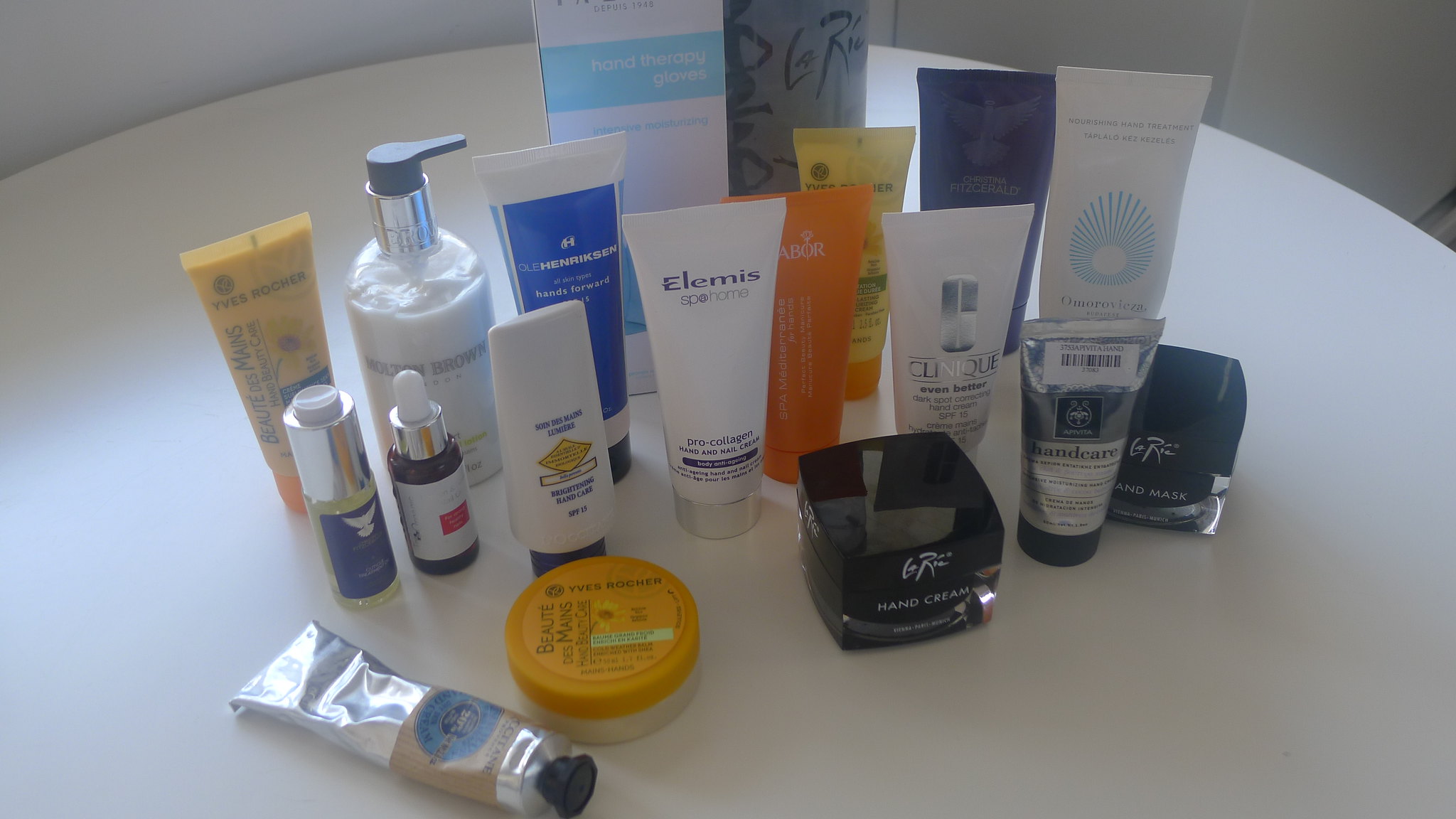A downward angled camera shot captures a room with pristine white walls and a round, white countertop adorned with various lotion products. From left to right, the assortment includes: a silver tube with a tan label featuring a blue circle, a small round jar of Yves Rocher cream, a tall silver and clear bottle with a blue label, a brown bottle with a white label and dropper, and a white bottle with a blue cap of hand lotion. Further along is a tube of Pro-Collagen Hand and Nail Cream from Spa Home, a green tube of lotion, a white tube of Clinique hand cream, and a silver tube of hand care. A square container of hand cream sits to one side, accompanied by a black container of hand mask. Just behind these items are a white tube of hand treatment, a blue tube from Christina Fitzgerald, a yellow tube, a gray tube, and, at the far left, a pair of hand therapy gloves.